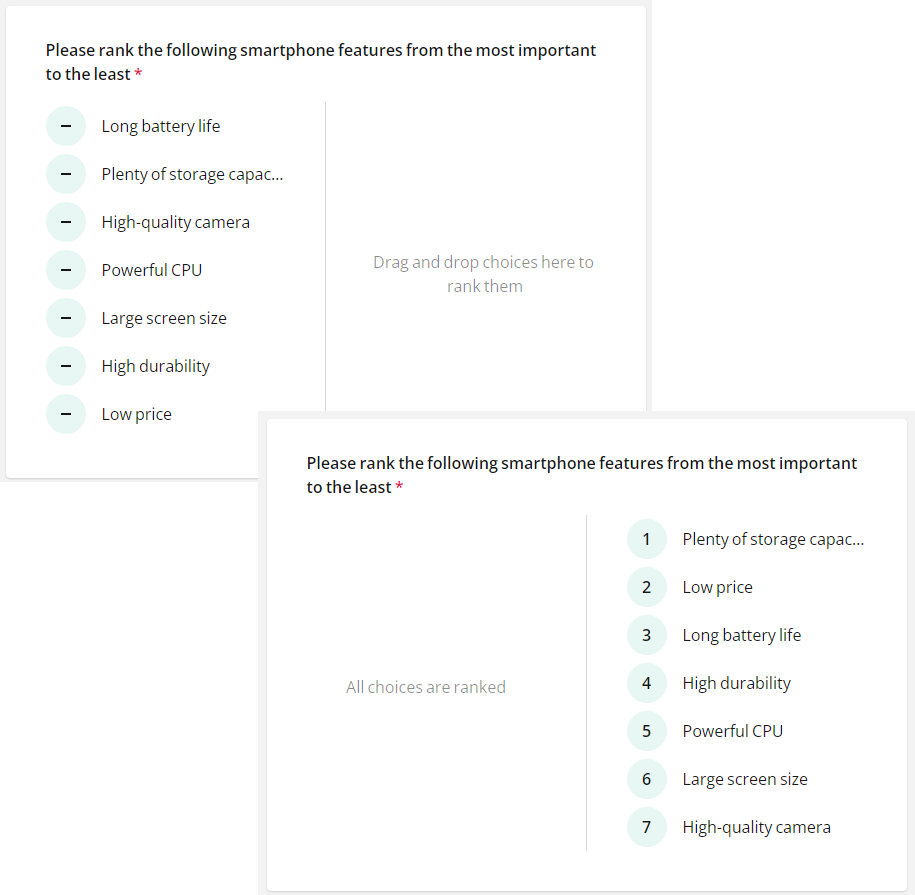The image portrays two boxes with text inside. Both boxes are nearly identical in composition and content.

In the top box, the text reads, "Please rank the following smartphone features from the most important to the least important." A small gray vertical line separates two sections within the box. The left section instructs, "Drag and drop choices here to rank them," while the right section shows a list of items accompanied by slightly blue circles containing small lines. The bottom part of this first box is obscured by the second box below it.

In the second box, the text also states, "Please rank the following smartphone features from the most important to the least important." Unlike the first box, here the items in the list are arranged and numbered from 1 to 7.

Both sections are centered around the task of ranking smartphone features, with the only visible difference being the inclusion of numerical ordering in the second box's list.